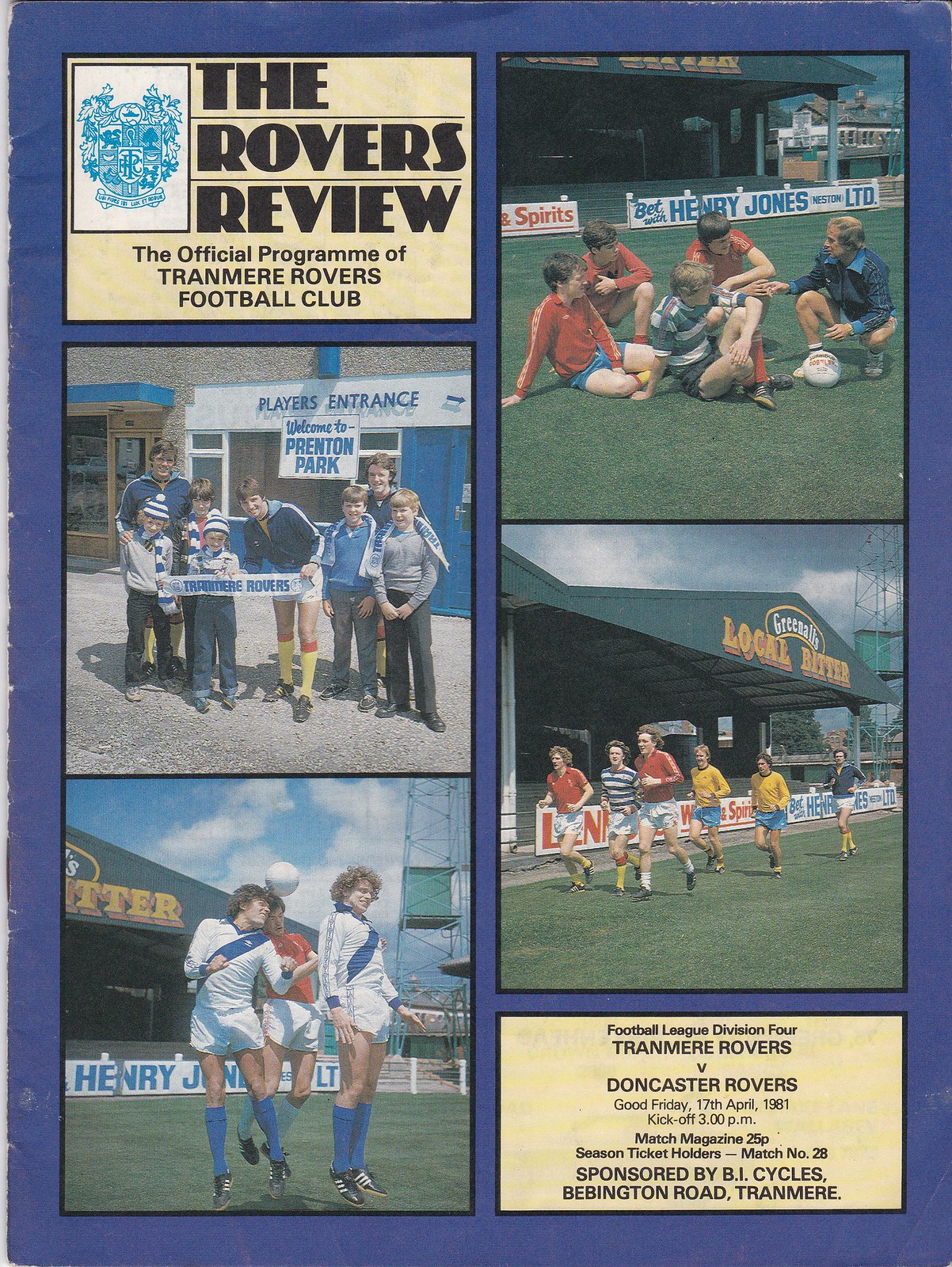The image is a cover of *The Rovers Review*, the official game day program of Tranmere Rovers Football Club, dated April 17, 1981. The magazine cover is predominantly blue with a tan box in the top left corner that reads "The Rovers Review" and features the club's insignia. It is noted that this is a special edition for a match against Doncaster Rovers in the Football League Division 4, scheduled for Good Friday, with a 3 pm kickoff.

The cover is adorned with four distinct photographs. The top left image shows a coach engaging in a discussion with four young boys, likely giving them a pep talk or instructions. The adjacent top right photo captures a group of children in front of the players' entrance, holding a ribbon with "Tranmere Rovers" emblazoned on it. This group includes four kids and three players.

On the bottom left, there is an action shot of three Tranmere Rovers players, dressed in their white and blue uniforms, with one of them heading the ball on the field. The bottom right corner depicts six players running in formation, evidently captured during a training session or warm-up drill.

Notably, the cover also mentions specific details about the match day, including the price of the magazine at 25 pence, its identification as match number 28 for season ticket holders, and sponsorship by B.I. Cycles, Bebington Road, Tranmere.